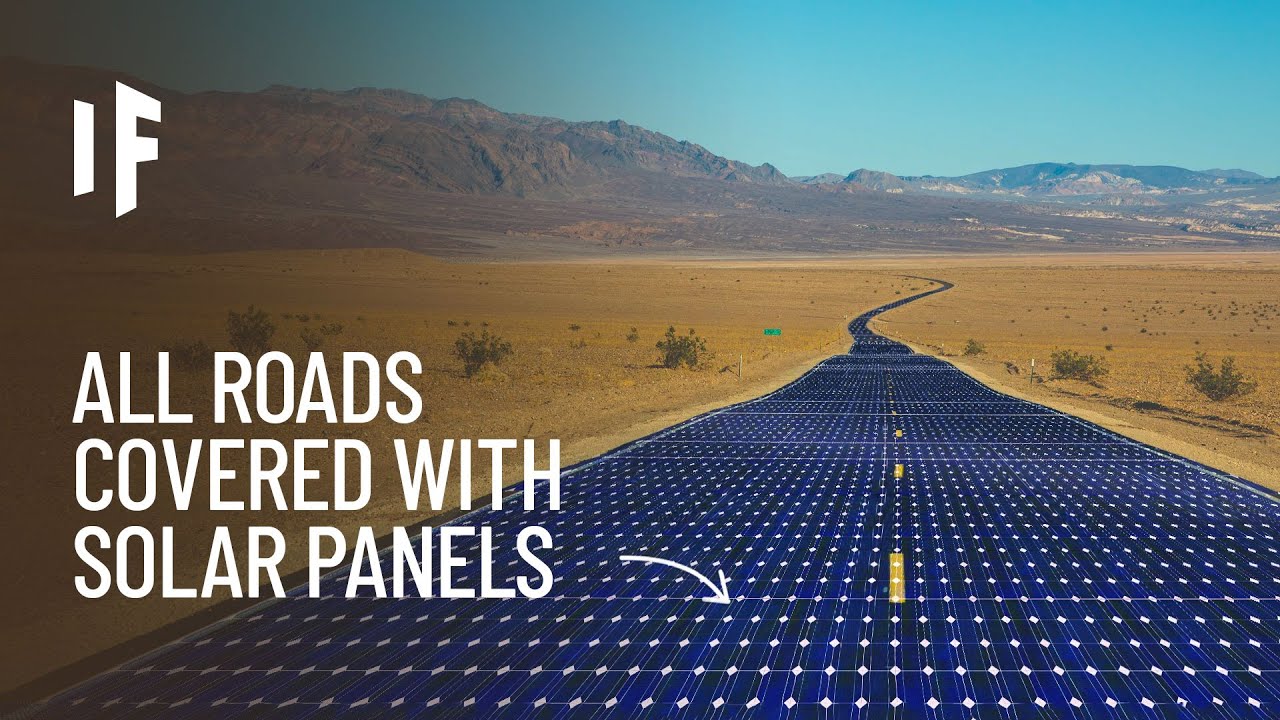The image is a rectangular, 3D proof-of-concept rendering showcasing a solar panel-covered road that stretches from the bottom right corner, extending into the distant horizon where it eventually disappears. The road is designed with tiny solar panels interconnected by white diamond shapes, and a yellow dotted line runs through its center. It traverses a flat, arid landscape characterized by dark yellow grass and the occasional small, stunted bush. The backdrop features distant brown mountains under a light blue sky. Imposed over the image is white text reading "IF all roads covered with solar panels," accompanied by a white arrow pointing towards the solar panel-covered road, suggesting a futuristic, eco-friendly infrastructure concept.